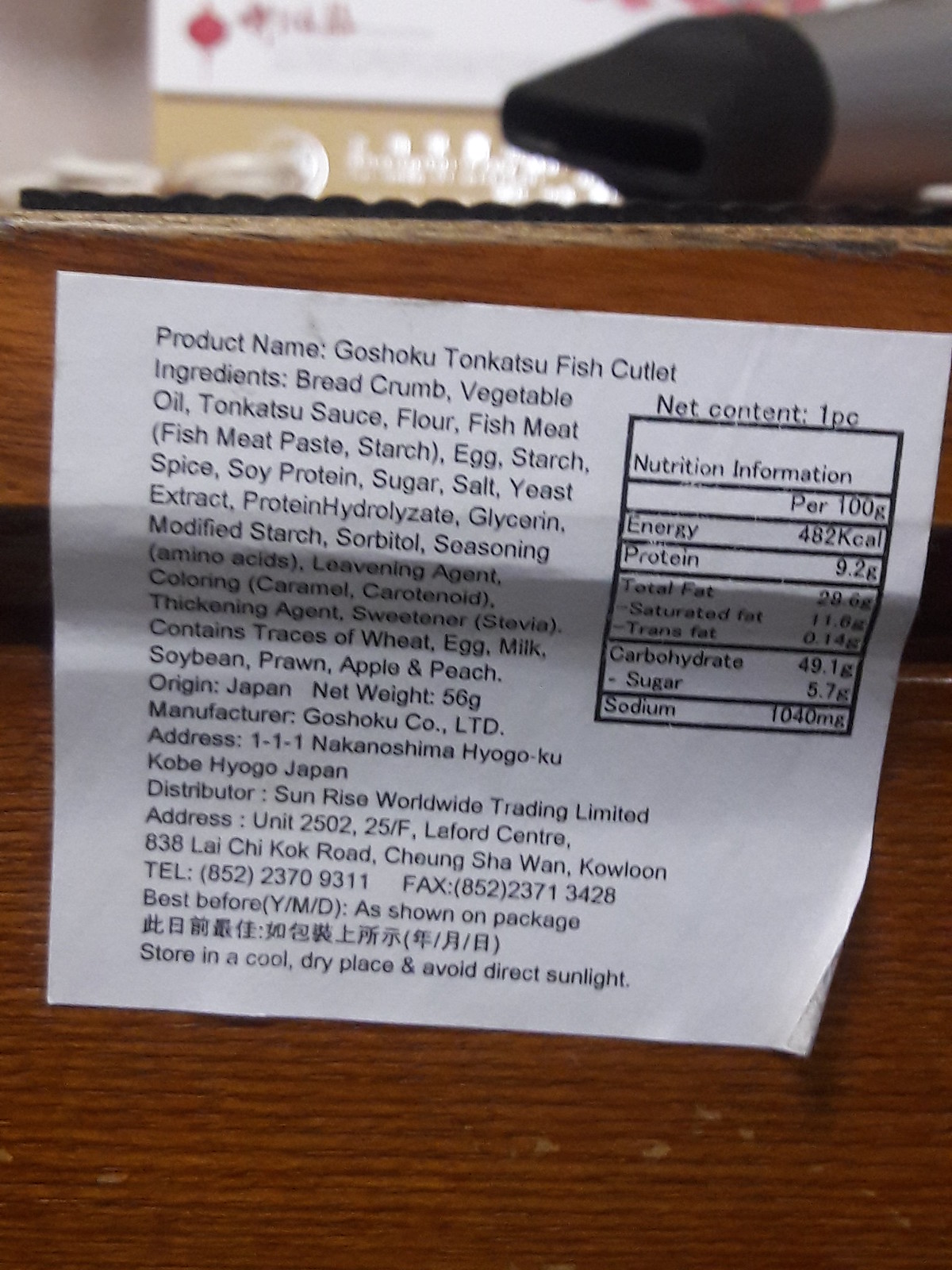The image shows an information sheet for a food product, identified as the Goshoku Tonkatsu Fish Cutlet, affixed to a wooden box. The label displays crucial information in black font, including the product name, ingredients list, manufacturer and country of origin details, various legal information, and a chart of nutrition facts highlighting calories, protein, fat, carbohydrates, and sodium content. The white label juts slightly over the lip of the wooden surface to which it is attached. The wooden box occupies most of the background, with a black nozzle lying on top of it and hints of another box with Asian characters visible. The label also includes a best-before date and storage instructions, advising to store in a cool, dry place and avoid direct sunlight.